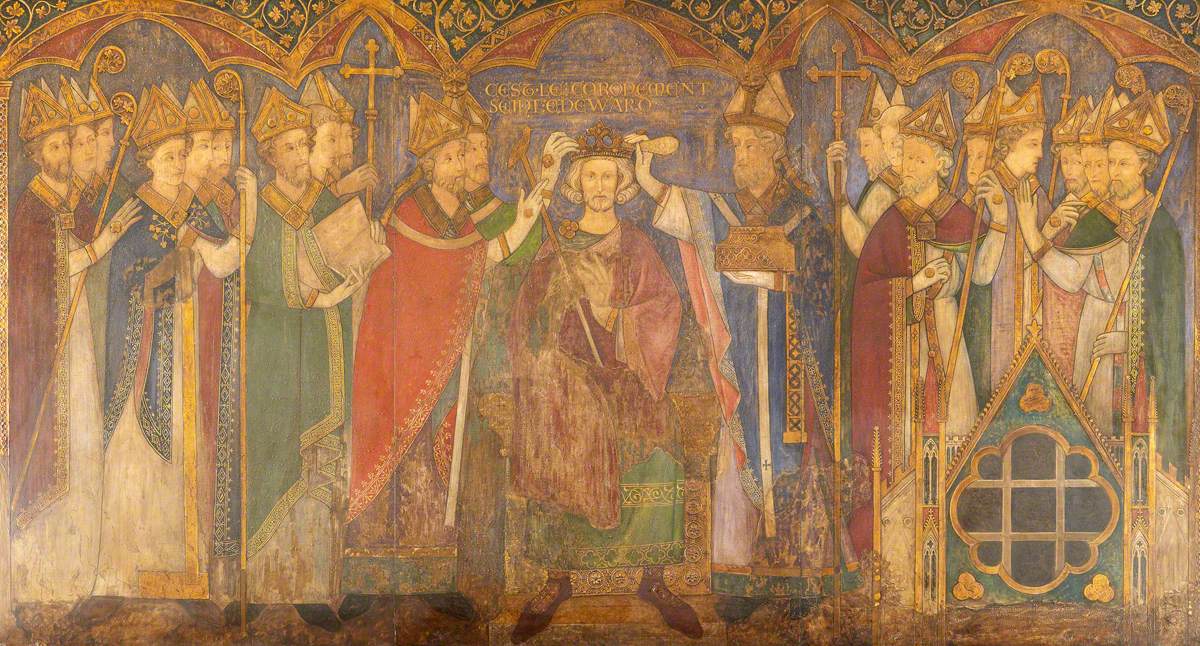This detailed artwork, possibly a watercolor or oil-based painting, presents a central figure who appears to be either a king or a high-ranking religious individual seated on a golden throne with a green bottom robe and a pink top. This central person is honored in the scene, surrounded by men who look like bishops or Apostles, recognizable by their ceremonial hats and staffs, some adorned with crosses. The array of colors in their robes includes vibrant reds, blues, greens, and purples. Above the seated figure, there is indecipherable yellow text, possibly in Latin. The scene appears to be set against a backdrop of gold and purple decorations, indicating a religious or royal setting. The painting, which could be part of a mural, shows signs of age, with weathering and fading impacting the visibility of certain details. On the periphery, clusters of men observe the central figure, some presenting crowns, suggested by their solemn gestures, while others on the far ends seem engaged in their own discussions, exhibiting either reverence or skepticism. Overall, the image conveys a highly ceremonial moment, rich in religious symbolism and regalia.